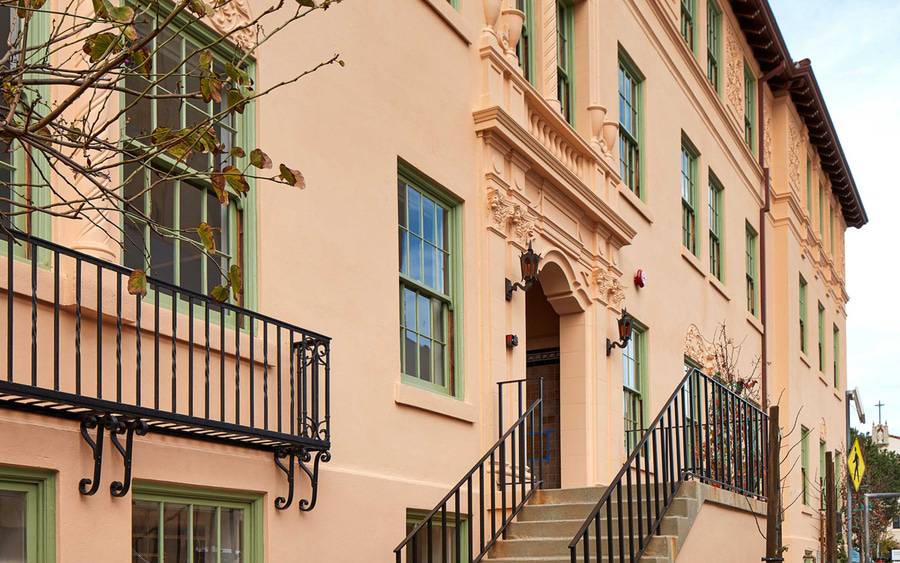This photograph captures a large, peach-colored, stucco building that boasts Victorian-style architecture, possibly an apartment building. The imposing structure, at least four stories tall and possibly including a basement level with street-level windows, is accentuated by ornate stonework, including pillars and carvings around the main entrance. The entrance, located on the second story, is reached via concrete stairs with black wrought iron railings and flanked by two vintage streetlights. The front door is set within an open arch that leads to a vestibule.

The building is adorned with numerous rectangular windows framed in sage green or seafoam green, creating a striking contrast with the peach facade. A small wrought iron balcony, wide enough for one person, is positioned under the window nearest to the camera, adding a touch of elegance. Above the entrance, there is also a tiny balcony serving the second-story windows.

The setting includes a pedestrian crossing sign and a security camera, adding to the urban feel. In the background, a church with a visible cross on its roof is discernible, along with a barren tree, suggesting a fall season. The presence of these elements suggests a picturesque neighborhood.